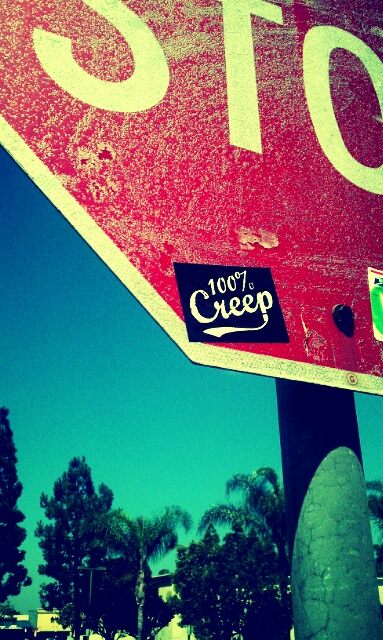This color photograph, taken in a narrow portrait orientation, features an extreme close-up of a weathered stop sign, focusing predominantly on its bottom left corner. The red of the sign displays signs of neglect, with a dingy buildup and streaks of white speckles marring its surface. Visible are portions of the letters "S," "T," and "O," while the "P" is completely out of frame. A black sticker with white lettering, reading "100% creep," is affixed to the bottom corner; the word "creep" features a metallic-like finish and an underlining swash, adding a distinctive flair. The background reveals a gradient sky transitioning from aqua to dark blue, suggesting either dusk or a filter effect, along with the tops of dark green trees and distant building outlines. The stop sign casts a shadow on its mounting pole, which is visible on the bottom right. The overall style of this image is photographic representationalism, capturing real-life details with a gritty, textured aesthetic.